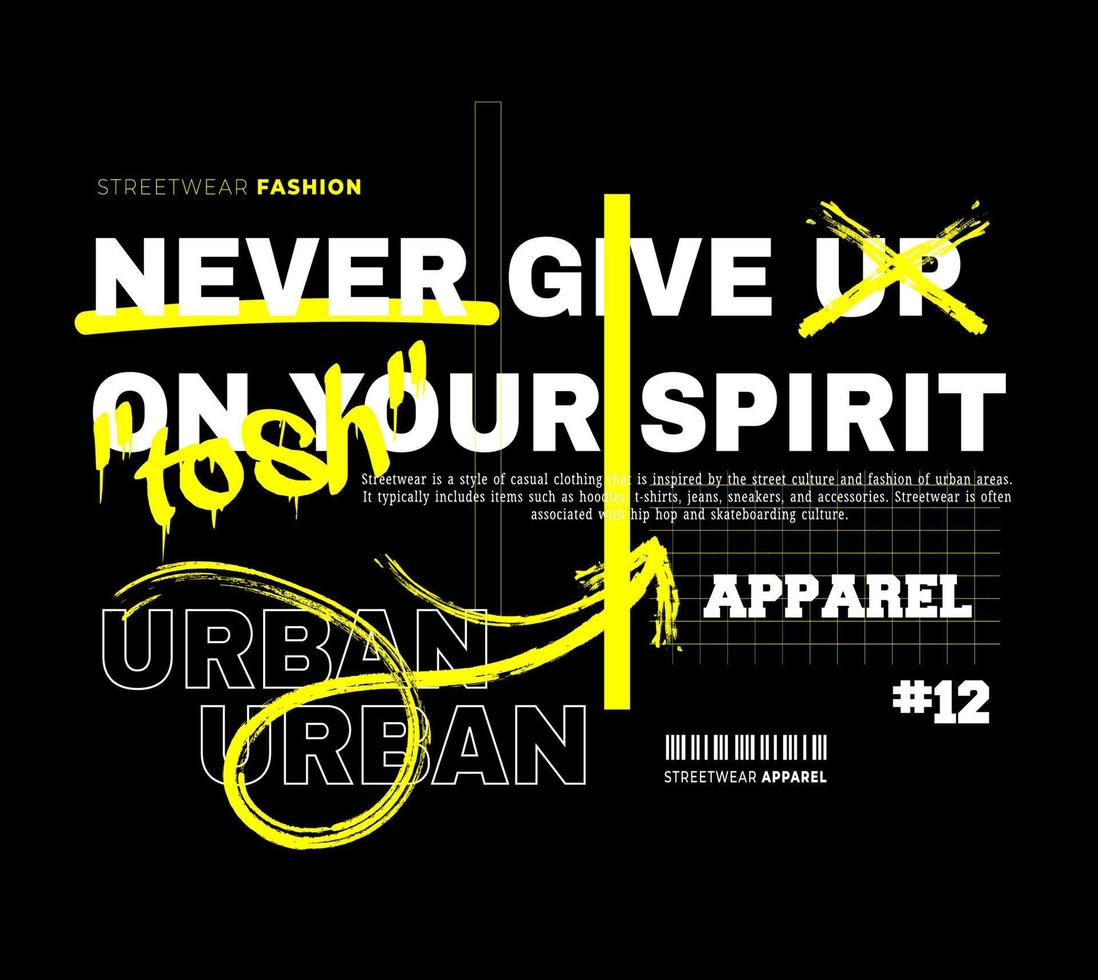This digital illustration serves as a striking advertisement set against a sleek black background. It features bold white and vivid yellow text, intricately layered in various fonts and styles to create a dynamic visual effect. The central message, "Streetwear Fashion: Never Give Up On Your Spirit," encapsulates the essence of streetwear's rebellious and resilient culture. A detailed, elongated paragraph further explores the unique style and cultural significance of streetwear. Additionally, a barcode-inspired graphic, labeled "Streetwear Apparel," adds an edgy, contemporary touch to the composition.